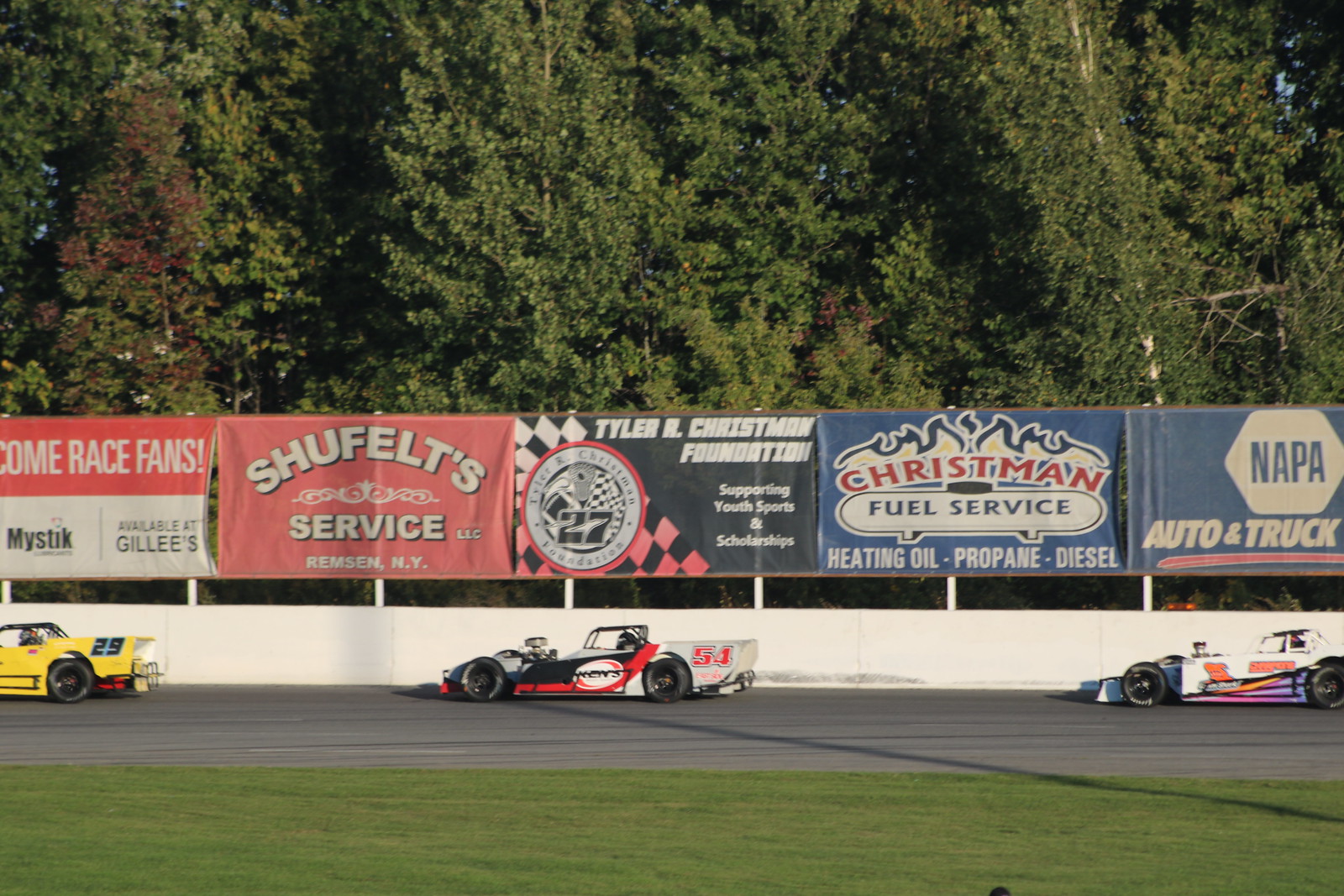The image captures an outdoor racetrack scene, framed by a lush green grass area in the foreground and surrounded by tall leafy trees in the background. In the middle of the gray asphalt track, three stock cars are racing. The car in the center, numbered 54, is a striking blend of gray, black, and red, with its driver visible, protected by a black roll cage. Ahead of it, the yellow car with bold black number 29 is slightly in the lead, while trailing behind is a white car accented with orange and purple. All three vehicles feature large, prominent front wheels, a characteristic of stock cars.

Encircling the track is a cement barrier lined with vibrant advertising banners. Notable signs include promotions for Napa Auto and Truck, Christman Full Service Heating Oil, Propane Diesel, and Tyler R. Christman Foundation, among others, adding splashes of red, blue, and white to the scene. The signage provides essential services and community support messages, enhancing the local racing culture backdrop. The vivid greenery of the trees adds a serene touch to the dynamic and busy racetrack environment.